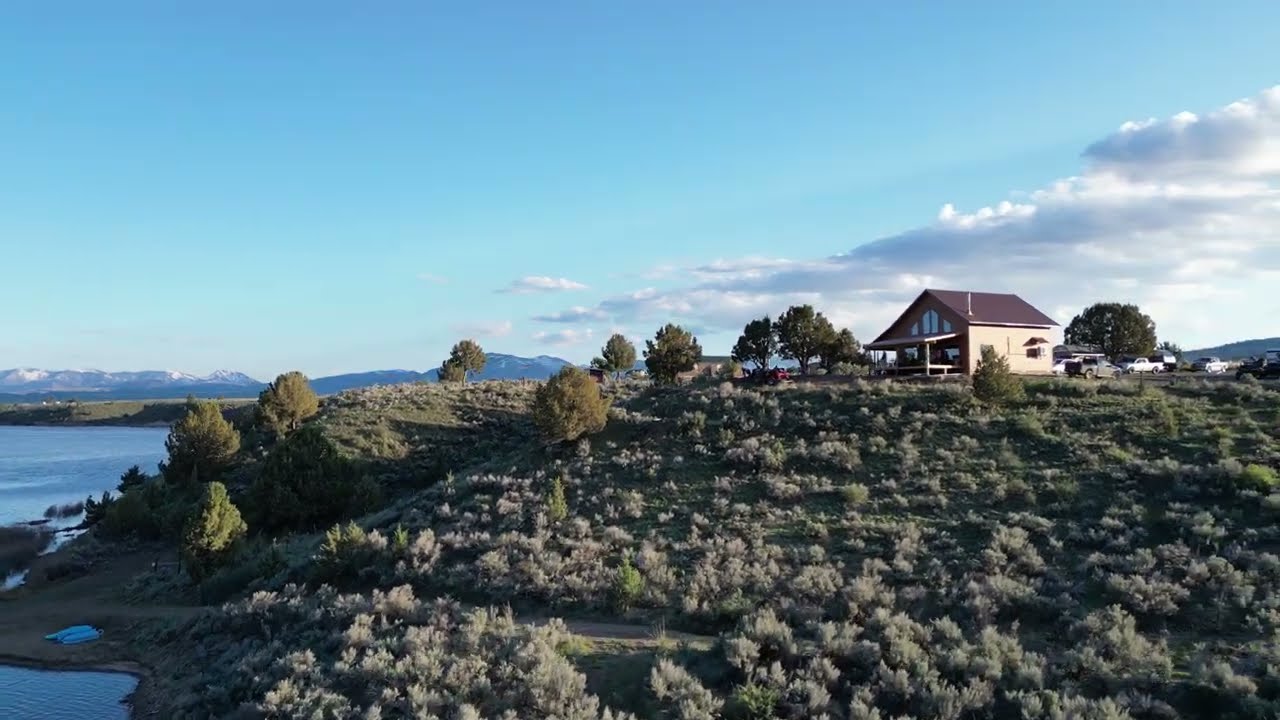A picturesque outdoor scene captures a small house perched atop a hill, overlooking a serene body of water. The house, which could be a country farmhouse or a small restaurant, features a reddish-brown roof and large windows facing the water. The siding of the house is a whitish color, adding a quaint charm to its appearance. Numerous pickup trucks are parked to the side and behind the house, indicating activity. The landscape is lush with green grass, bushes, and several trees, including one prominent tree behind the house. In the background, a range of mountains, some with snow-capped peaks, stretches across the horizon, enhancing the secluded and tranquil setting. The sky is predominantly clear blue with a few clouds, providing a stunning backdrop to this idyllic hilltop dwelling.